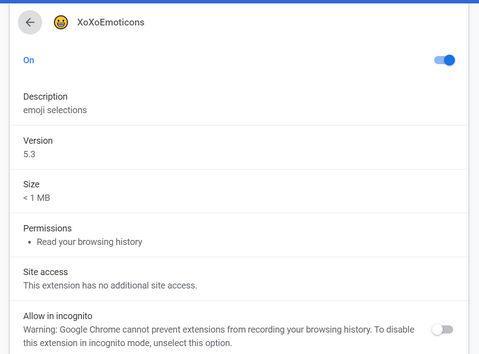The image shows a webpage with a clean, white background. At the very top, a thin blue line extends horizontally from left to right. Immediately below this line, there is a circular icon featuring an arrow pointing to the left. To the right of this icon, there is a small yellow smiley face.

Adjacent to the smiley face, it says "XOXO Emoticons" in a stylized format where the 'X's and 'E' are uppercase and the remaining letters are lowercase. Immediately to the right of this text, the word "ON" is displayed with a capital 'O' and lowercase 'n' in blue font. Towards the far right end of the screen, there is a blue toggle switch that is in the "on" position.

Below this section, there is a heading in small black print labeled "Description," with the subheading "Emoji Selections" underneath. A thin gray line separates this section from the next.

The subsequent section begins with the heading "Version," followed by the version number "5.3". Another thin gray line follows, leading to the next heading, which is "Size" with a capital 'S'. Below this, the size is indicated as "< 1MB," with "MB" capitalized. Another thin gray line marks the end of this section.